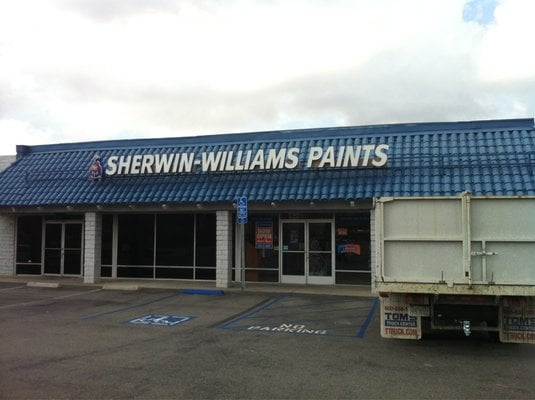A photograph captures the storefront and parking lot of a Sherwin-Williams Paints store. The store features a distinctive blue roof adorned with curved, Spanish-style shingles. Prominently displayed above the entrance is the Sherwin-Williams Paints logo. The storefront is characterized by extensive glass windows and includes two sets of double glass doors, one positioned to the right and the other to the left.

In the parking lot, at least two open spaces are visible alongside a designated handicapped space. Directly in front of the main entrance is an area marked for no parking. Adjacent to this no-parking zone is a large truck with a substantial trailer, identifiable only by partial advertising on its mud flaps reading "Tom's," indicating a trucking service.

The image also features an overcast sky, with thick clouds allowing only a hint of blue to peek through, creating a subdued daylight atmosphere.